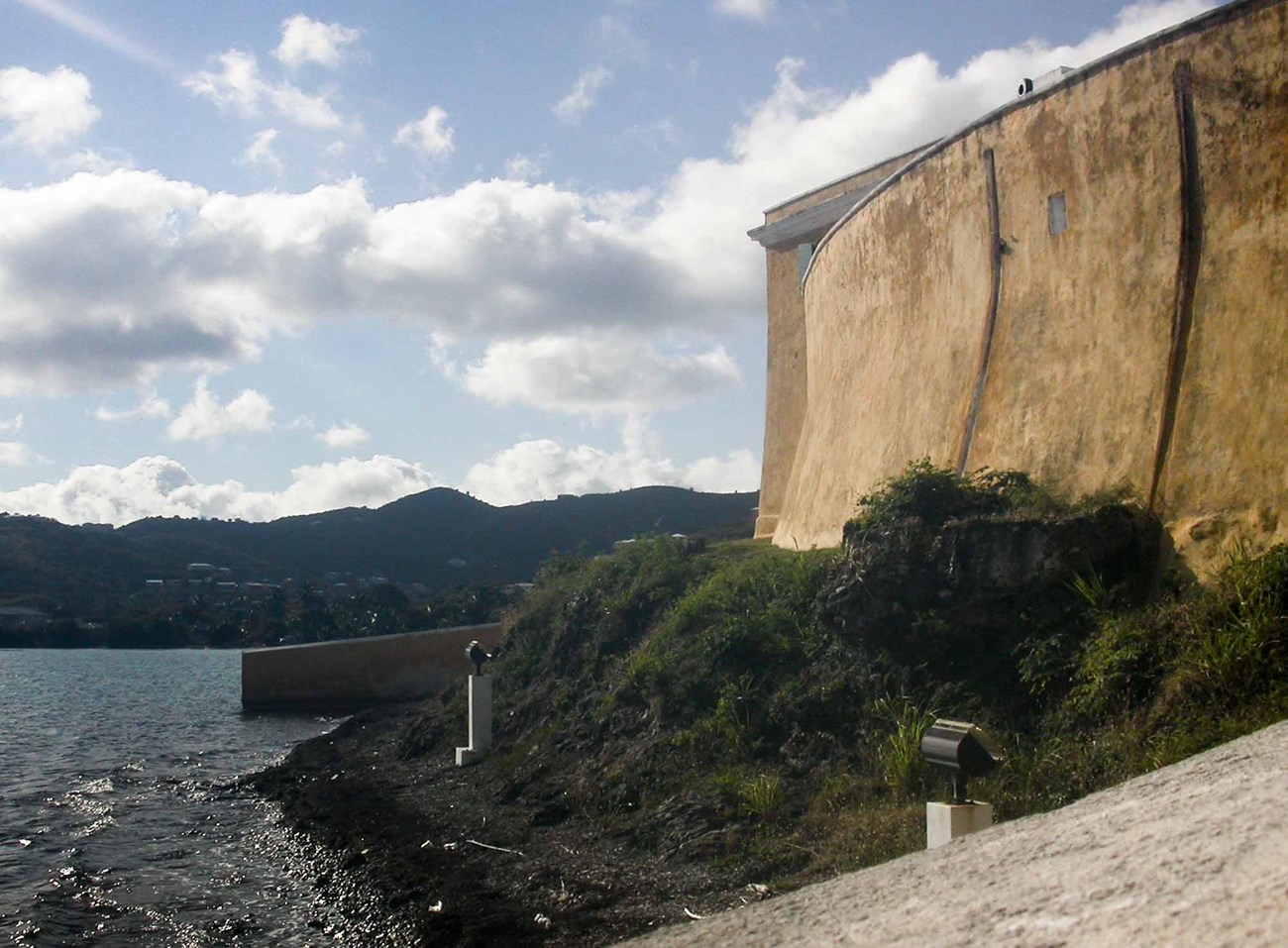The image features a large, brownish-tan dam with an angled, half-circle shape, which slopes down into a small, grassy island designed to hold the bank and prevent erosion. Standing atop the dam are several people, gazing over its edge. At the base of the grassy mound are two black spotlights mounted on cement, illuminating the dam for nighttime visibility. The expansive background showcases a mountain range covered in green trees, a town with predominantly white buildings, and a serene lake with grayish-blue water. The sky above is a light blue, dotted with fluffy white and gray clouds. The scene is framed by additional cement structures on either side, adding more depth to the landscape.